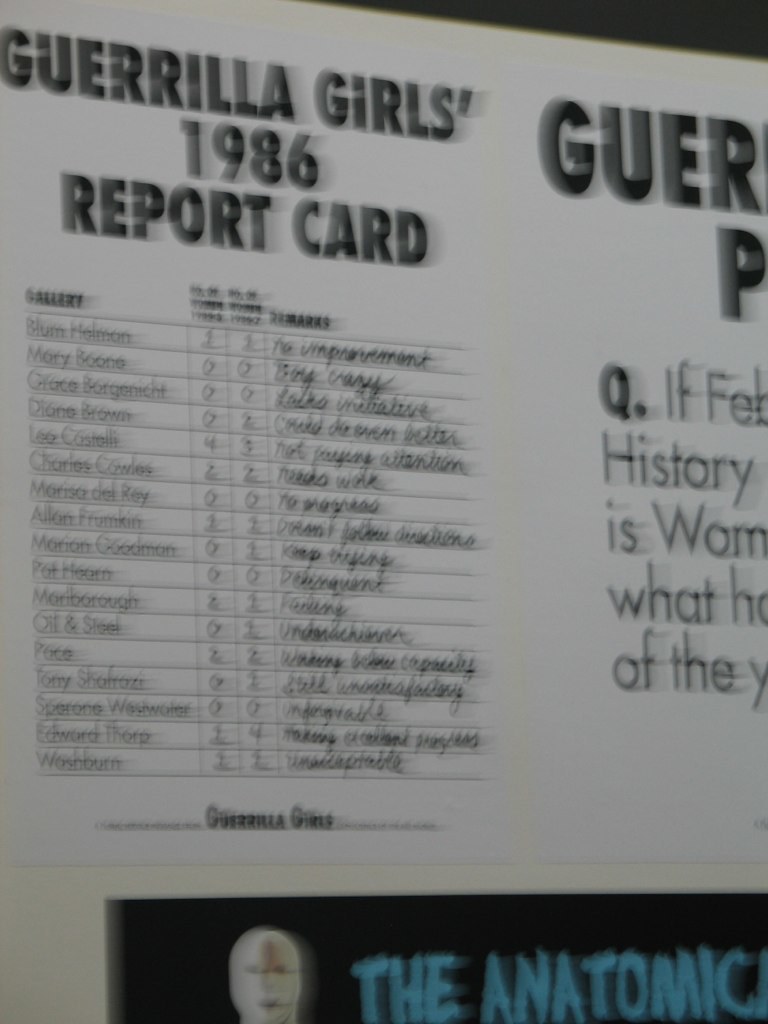This photograph, albeit blurry, is a depiction of a poster titled "Guerrilla Girls 1986 Report Card" in bold, all-caps black letters on a white background. Below the title, there are four columns: the gallery column listing approximately 20 names vertically, each followed by a grade, and then a remarks column featuring handwritten comments such as "no improvement," "underachievement," "belligerent," "failing," "underachiever," and "unforgivable." On the right side of the image, a partial text reads "G-U-E-R," followed by a "Q," and beneath it, an incomplete sentence starting with "If February history is woman, what...?" The lower part of the poster features the word "The Anatomic," with additional indecipherable letters following. The background seems to be a wall, and there is also an image of a man’s head, possibly wearing a mask, adding to the complex visual scene within this artwork by the Guerrilla Girls.